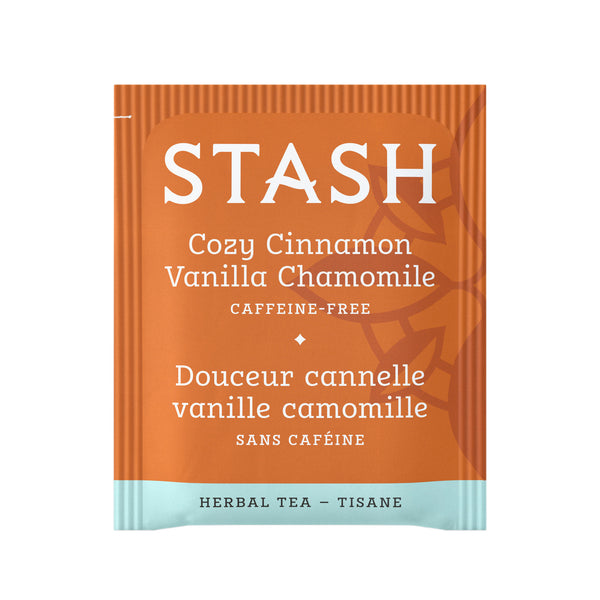This image showcases a Stash tea packet designed for Cozy Cinnamon Vanilla Chamomile, labeled as caffeine-free. The packaging is primarily a burnt orange or umber color, transitioning to a lighter aquamarine strip at the bottom which reads "Herbal Tea - Tisane" in black. The top center prominently displays the brand name "Stash" in large white letters. Below, in smaller white text, are the tea flavors "Cozy Cinnamon Vanilla Chamomile," along with a small white star, and a repetition of this information in French. The background features subtle darker orange designs resembling leaves in a circular pattern. The packet, intended for tear-open use, includes a faint white tear line at the top left for easy opening. The sides and top have subtle ridges, adding texture to the simple design against the white backdrop.